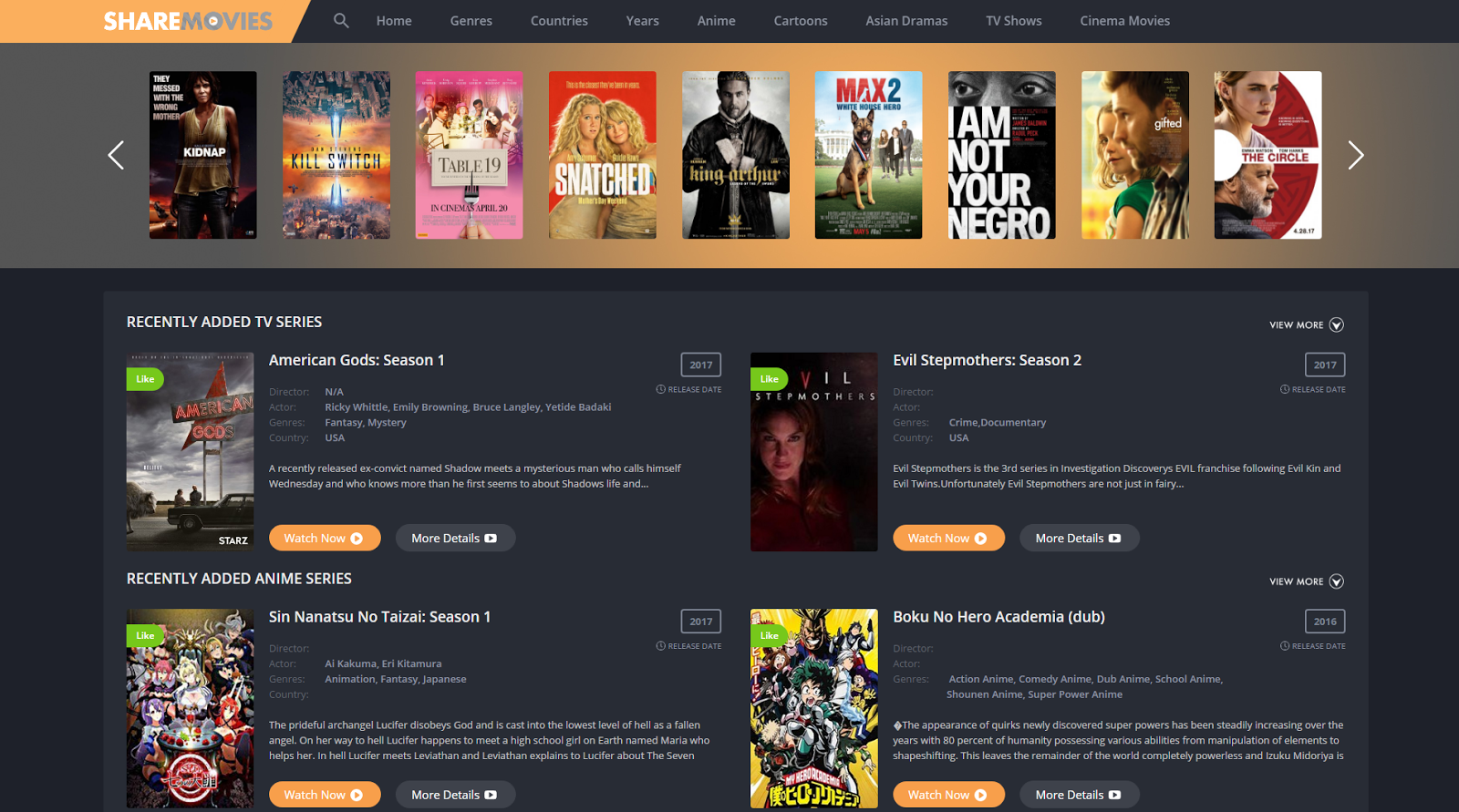This image showcases the homepage of a website called "Share Movies," prominently indicated in the upper left corner. Moving right from the logo, the navigation menu includes a search icon and categories such as Home, Genres, Countries, Years, Anime, Cartoons, Asian Dramas, TV Shows, and Cinema Movies, offering a broad selection of entertainment.

Directly below the main menu is a rotating carousel displaying nine movies: Max 2, I Am Not Your Negro, Gifted, The Circle, Table 19, Snatched, Kill Switch, and Kidnapper, among others. Arrows on either end allow users to scroll through these options, although there are no descriptions provided for the titles.

Below the carousel, the section titled "Recently Added TV Series" features four entries: "American Gods Season 1," "Evil Stepmother Season 2," "Boku no Hero Academia" (listed as dubbed), and "Sin Nenetsu no Teizai Season 1" (a title of apparent Asian origin). Each entry includes information such as the director (not available in this case), genres, and countries of origin.

While the legality of the website is uncertain, it is well-organized and visually appealing.